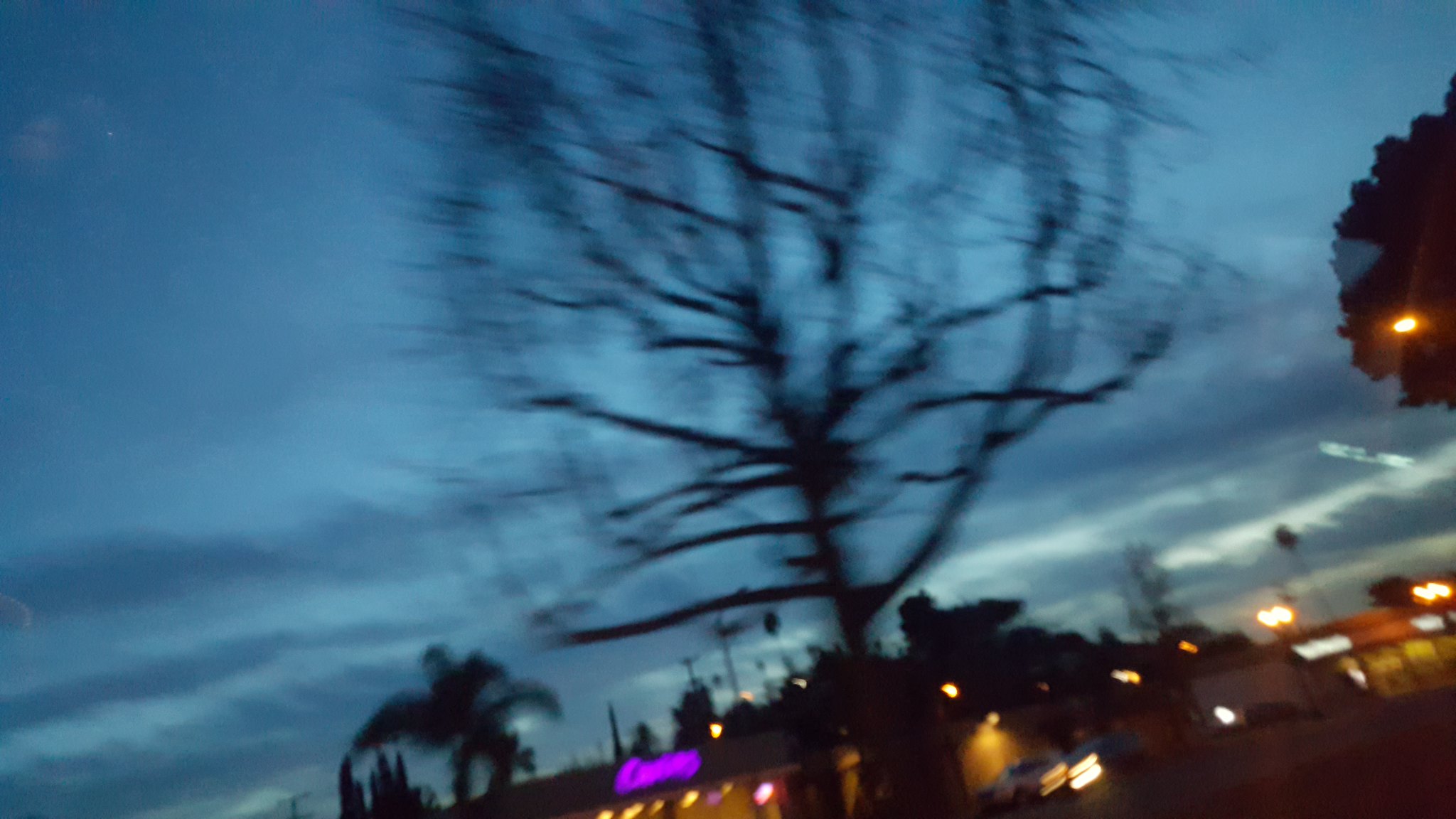A blurry image depicts a predominantly cloudy sky transitioning from light to dark blue. The sky covers the majority of the frame and is peppered with gray clouds. In the center of the image stands a large tree with branches extending both left and right. The top right corner of the image shows a portion of another tree jutting into the frame. Several streetlights glow softly throughout the scene. At the bottom center, a storefront sign illuminated in purple light adds a splash of color to the otherwise muted backdrop. Despite the lack of clarity, the scene captures a moody, atmospheric setting.